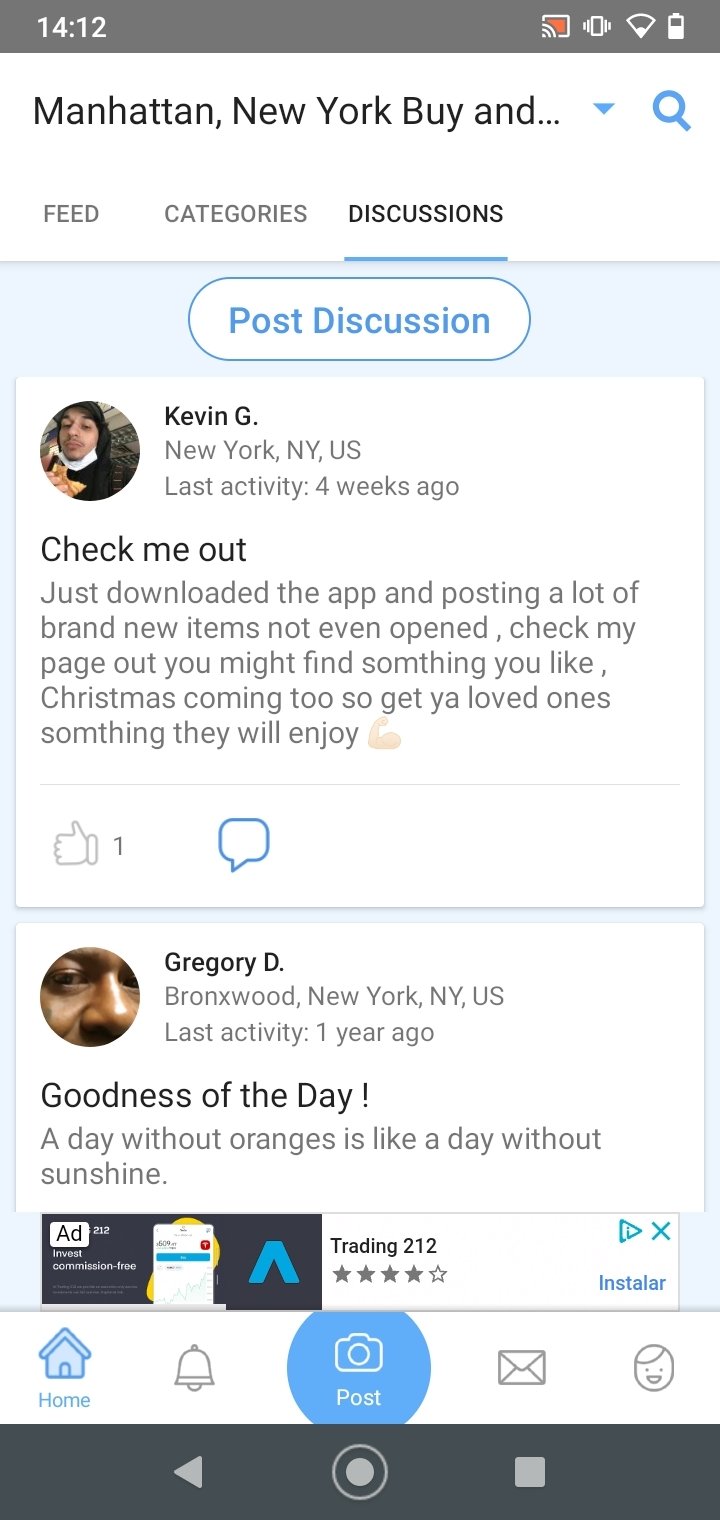The screenshot displays a cell phone screen with a dark gray border at the top. The time "14:12" is shown in the upper left corner. Below this, the text "Manhattan, New York, by..." is written in black. Beneath this section, there are three tabs labeled "Feed," "Category," and "Discussions," with "Discussions" highlighted. Under the "Discussions" tab, there is a blue-bordered section titled "Post Discussions."

To the left of this blue-bordered section is a circular icon featuring a photograph of a person. Next to this icon, the text reads, "Kevin G., New York, New York, U.S." and "Last activity four weeks ago." In bold text, it states, "Check me out." This is followed by the message, "Just downloaded the app and posting a lot of brand new items not even opened. Check my page out, you might find something you like. Christmas coming too, so get your loved ones something they will enjoy."

Below Kevin G.'s post, there is an image of a thumbs-up icon accompanied by the number "1" and a speech bubble icon. Below this, on the left side, is another circular icon with a close-up image of a different person's face. Next to this icon, the text reads, "Gregory D., Bronxwood, New York, New York, U.S." and "Last activity one year ago." In bold text, it states, "Goodness of the day," and the message, "A day without oranges is like a day without sunshine."

Below Gregory D.'s post are a couple of ads. At the bottom of the screen, there are icons depicting a house, a bell, a camera, an envelope, and a person. Along the dark gray bottom border, there are additional icons: an arrow pointing to the left, a circle with another circle inside it, and a square.